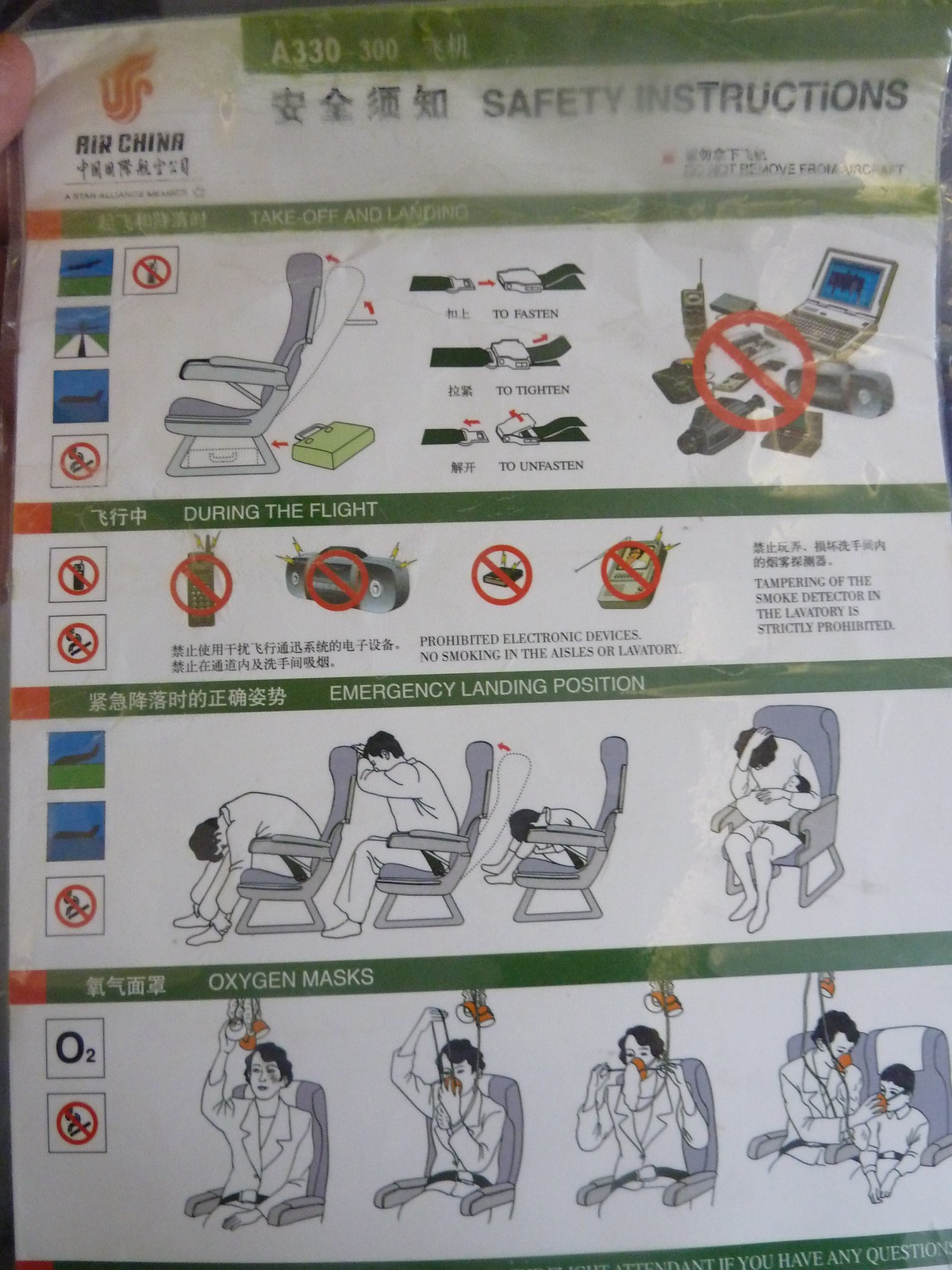This detailed image depicts a piece of paper labeled "Safety Instructions" for an Air China A330-300 aircraft, written in both English and Mandarin. The top section outlines the proper use of a seat belt, displaying how to fasten and unfasten it. Further down, a prohibition on electronic devices during takeoff and landing is emphasized, featuring symbols of banned devices such as computers, cell phones, cameras, and boom boxes. There's a red circle with a diagonal line through it over these items to reinforce the restriction. 

The instructions also detail safety measures during the flight, including a prohibition on smoking and the use of specific electronics like pagers and portable TVs. One section is dedicated to emergency landing positions, showing various crouching and bracing techniques, with illustrations including a woman and a child demonstrating the correct posture. Further instructions illustrate the deployment and proper usage of oxygen masks, again highlighting a model of an older woman assisting a smaller child. Overall, the safety instructions are clearly organized into four sections, ensuring passengers know how to stay safe and respond in case of an emergency.